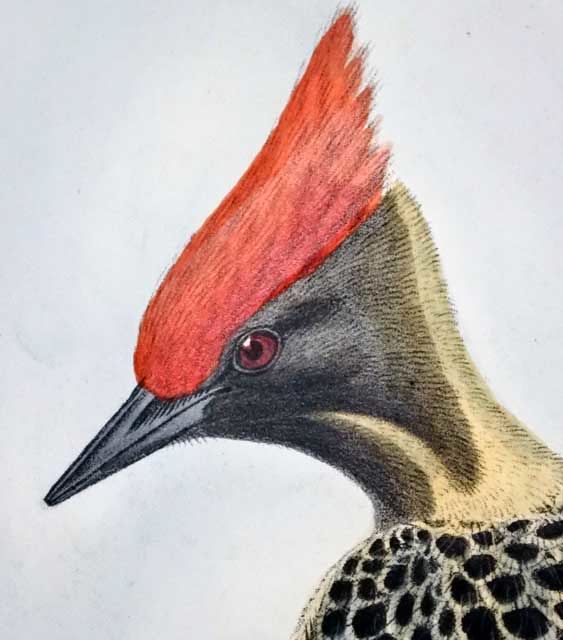The image is a highly detailed color sketch of a bird's head, closely zoomed in, giving it an almost painting-like appearance. The background is a light gray or white, resembling sketch paper or canvas. We see the bird from a side view, highlighting its intricate features. The bird's head is topped with vivid red feathers, transitioning to dark brown and black towards the face. The beak is black, and the eye is strikingly red with a black pupil, showcasing detailed irises and a glimmer of light. The neck is a light beige or tan color, which transitions into darker hues and is adorned with black and white feather patterns. These feather patterns extend slightly into the top part of the bird's wing, creating an impression of black scales or netting. This captivating representation, possibly rendered with colored pencils or pens, emphasizes the bird's vibrant coloration and textured plumage against the clean, monochromatic background.